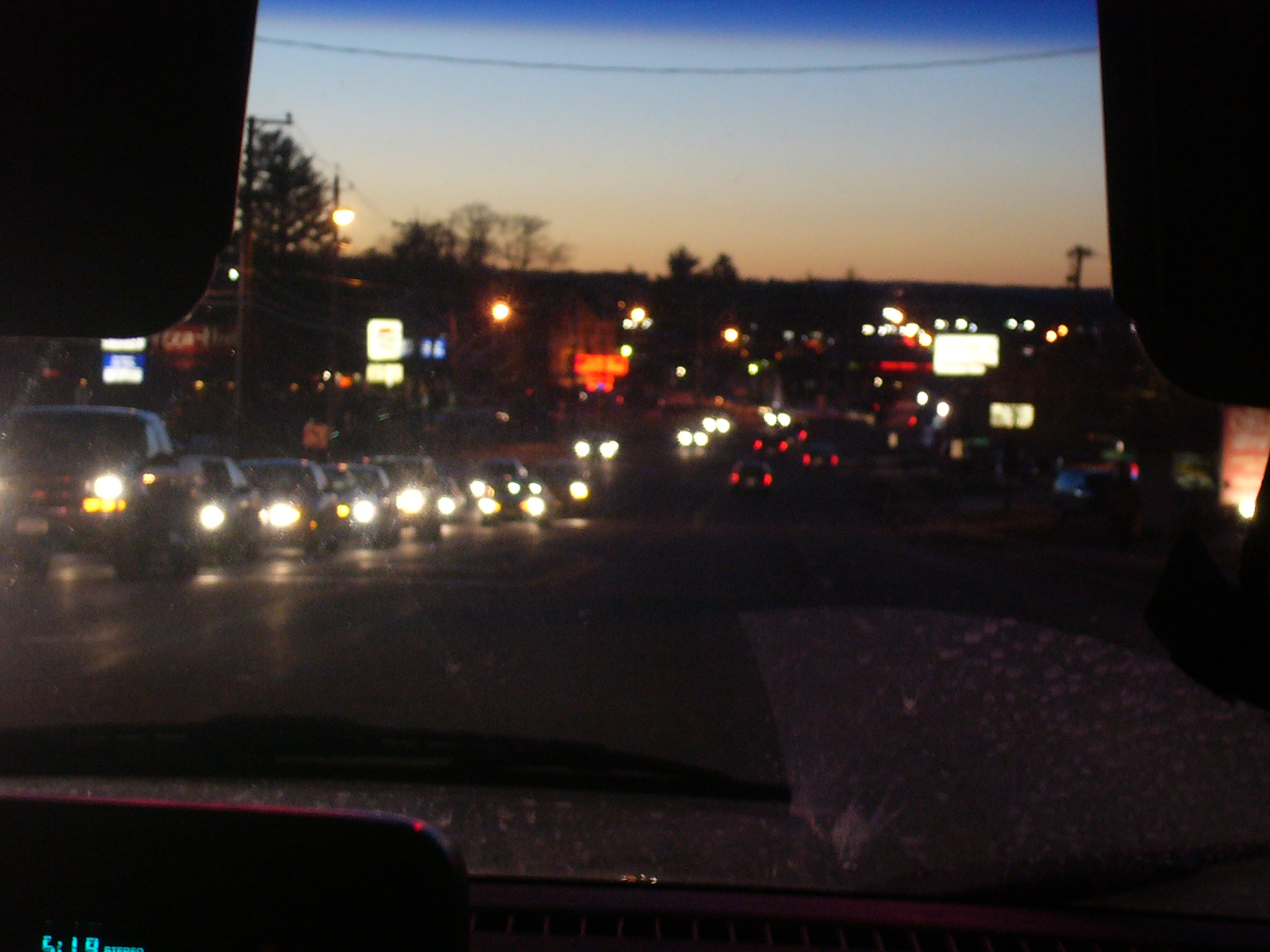This outdoor photograph, taken at dusk through the slightly scummy windshield of a vehicle, captures a nighttime scene just after sunset. The horizon, located about two-thirds up the image, is flat and transitions from a light purple to light blue to dark blue sky. In the foreground, a stream of approximately 10 to 12 oncoming cars with illuminated headlights travel towards the photographer in the left lane, while the right lane's traffic moves away into the background. The road is flanked on both sides by bright signs from various businesses, including notable orange and white ones, and street lamps illuminating the surroundings. On the left side, sparse leafless trees and a tall pine tree are visible. A portion of the car’s LED clock, displaying 5:19 p.m., is slightly cut off in the lower right corner, adding a faint hint of the car's dashboard to this dimly lit, slightly out-of-focus image.